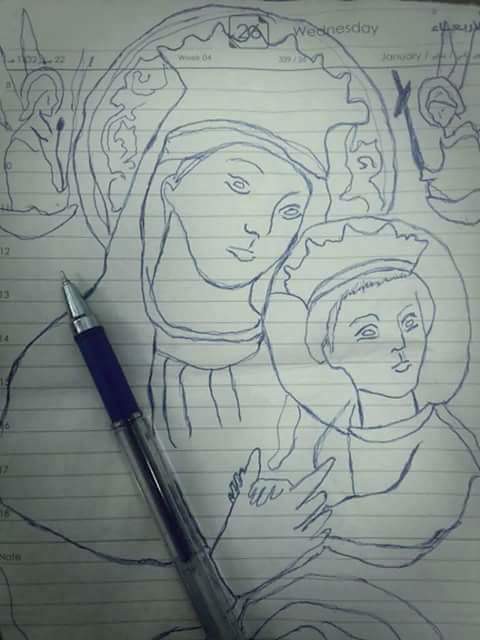The image depicts a detailed blue pen sketch on lined white notebook paper, likely from a day planner, with “Wednesday” and the date “26” written at the top. The drawing illustrates a central holy scene: a woman, possibly Mary, wearing an elaborate crown with a detailed halo, holding hands with a young boy, possibly a young Jesus, who also wears a crown and a halo. Surrounding them are angelic figures with wings and halos, with one angel holding a large cross. Both angels appear to be kneeling and praying. A blue pen, with its cap off, is resting vertically along the edge of the paper, overlapping the intricate sketch.